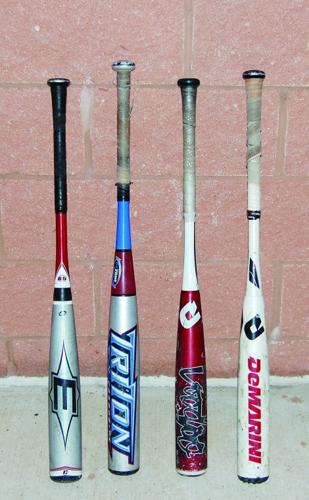This detailed color photograph in portrait orientation showcases four baseball bats leaning against a pinkish, reddish-brown block wall with a gray concrete ground beneath them. The bats, varying in size, shape, and graphics, are arranged vertically from left to right. 

The first bat, an Easton, features a gray barrel that narrows into a red section, paired with a black handle and knob. The second bat is a Triton with a prominently dirty white handle, a light blue stem, and a red circle, concluding with a gray barrel marked "Triton" in gray and blue. The third bat is a DiMarini Voodoo, characterized by a black knob, white grip tape, and a red section displaying "Voodoo" in black and the DiMarini logo - a white 'D'. The final bat also sports a black knob and white grip tape, complemented by a solid white barrel with "DiMarini" in red and a black 'D' logo at the end.